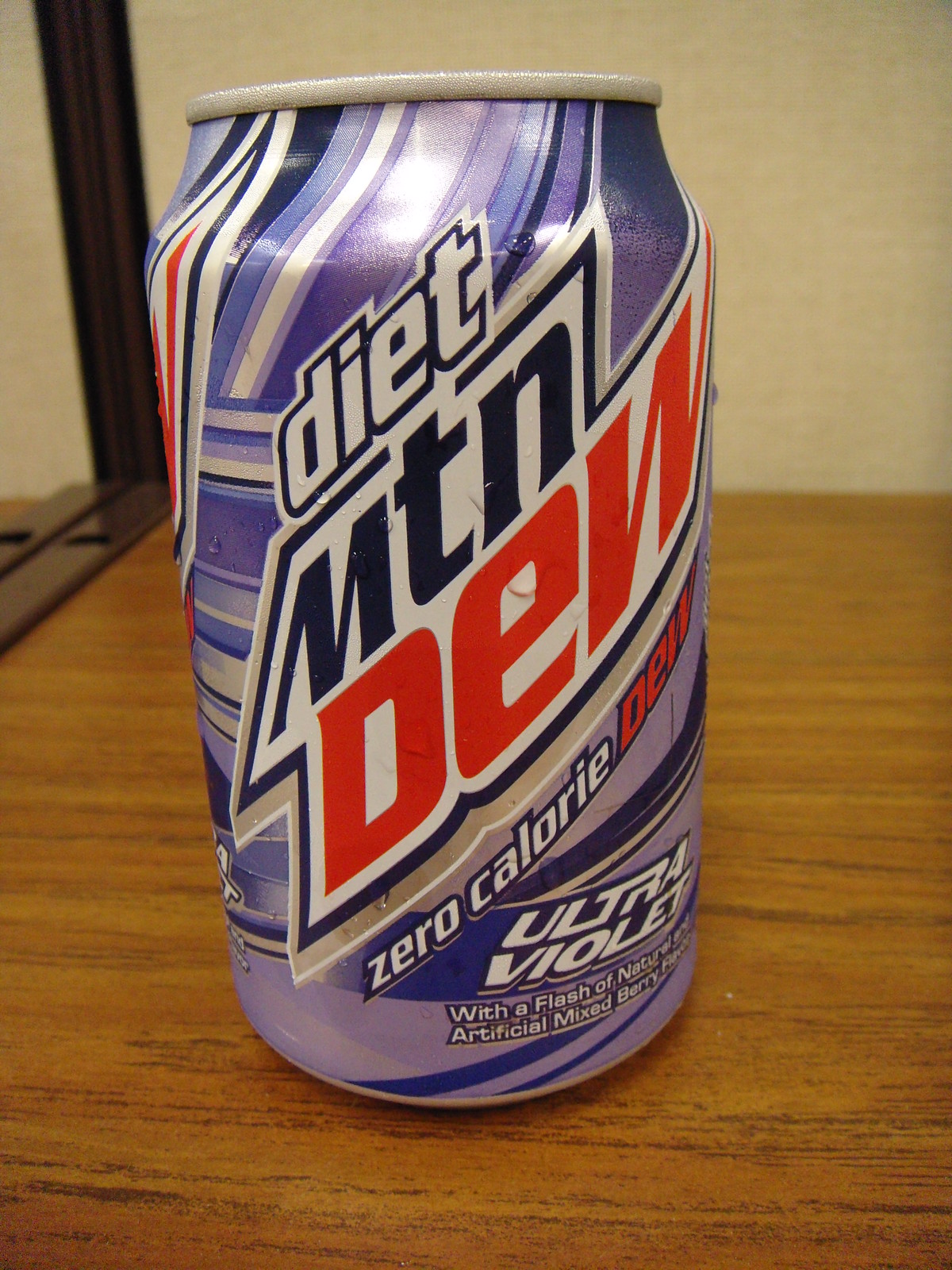The image shows a can of Diet Mountain Dew Ultraviolet prominently placed on a hardwood desk surface. The desk, possibly featuring brown brackets at the corners, appears to be positioned next to either a mirror or another similar desk, which is noticeable but partly cropped out along the left edge of the frame. A dark-toned seam can be seen to the left, likely attaching two partitions that look fabric-covered in light gray, as opposed to being solid walls.

The soda can itself boasts a striking design with blue, silver, white, and red colors. The label clearly reads "Diet Mountain Dew, Zero Calorie Dew, Ultraviolet," highlighting its mixed berry flavor with both natural and artificial ingredients.